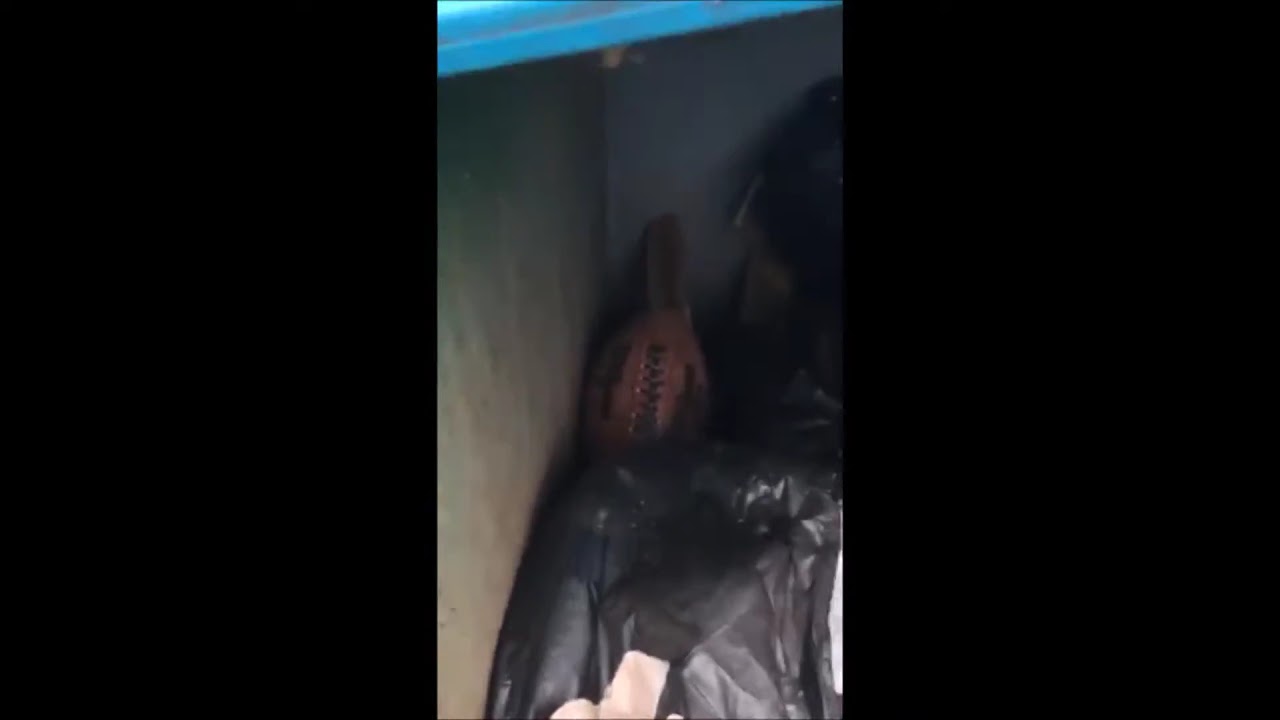The photograph depicts a somewhat cluttered and dimly lit scene viewed within a vertical rectangle taking up approximately one-third of the image, framed by black margins on either side. Dominating the top portion is a diagonal light blue bar, possibly indicative of a shelf, suggesting the setting might be a locker, closet, or other enclosed space. The back and left walls are gray, contributing to the overall low-light ambiance. Central to the image, there is a black plastic material, likely a bag or jacket, resting in the bottom half, and above it sits a distinct football with visible stitching. The coloring, mostly gray, black, brown, white, and light blue, makes object identification challenging. The scene is set indoors, possibly in a dark room, or, as one interpretation suggests, inside a teal green dumpster containing black bags and a torn football with exposed insides.